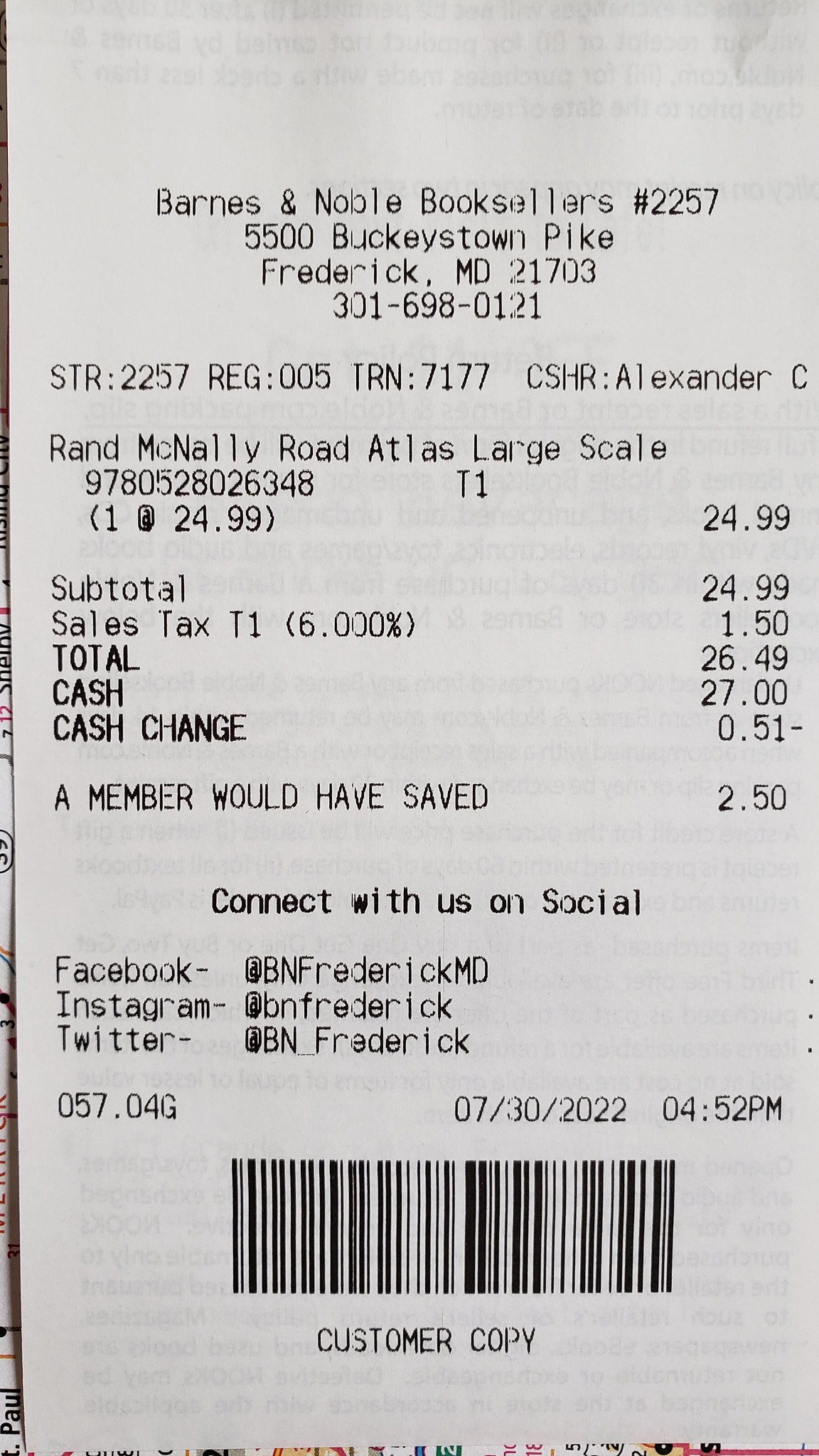This image is a close-up, portrait-oriented receipt from Barnes & Noble booksellers, located at 5500 Buckeystown Pike, Frederick, MD 21703. The receipt, which features a white background with black text, details the purchase of a Rand McNally Road Atlas, Large Scale for $24.99. With the addition of $1.50 in sales tax, the total amount comes to $26.49. The customer paid $27.00 in cash and received $0.51 in change. Noted on the receipt, members would have saved $2.50 on this purchase. Additional information includes the cashier's name, Alexander C., and contact details for the store (phone number: 301-698-0121). At the bottom, the receipt prompts customers to connect on social media platforms like Facebook, Instagram, and Twitter, and it is marked as a "customer copy." A barcode and timestamp are also present, further authenticating the retail receipt from Barnes & Noble booksellers.